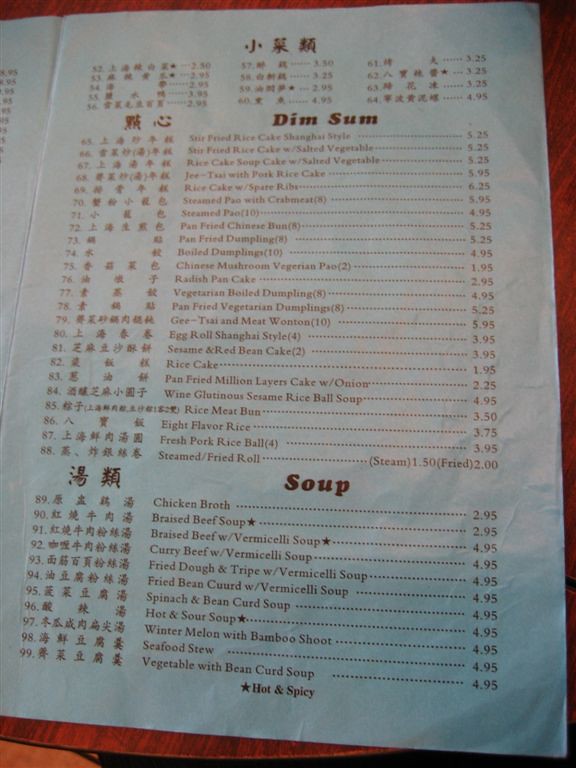This menu, presented on white paper with dark red text, features both Asian characters and English descriptions. At the top, Asian characters are accompanied by numerical values. The left side of the menu lists numbers ranging from 52 to 99, each accompanied by corresponding Asian characters. 

Under the "Dim Sum" header, a variety of items and their prices are listed:
- Stir-fried cake, Shanghai style – $5.25
- Stir-fried rice cake with salted vegetables – $5.25
- Rice cake soup with salted vegetables – $5.25
- Gisao beef with pork rice cake – $5.95
- Rice cake with spare ribs – $6.25
- Steamed pao with crab meat – $5.95
- Steamed pao – $4.95
- Pan-fried Chinese bun – $5.25
- Pan-fried dumplings – $5.25
- Boiled dumplings – $4.95
- Chinese mushroom Chinese pao – $1.95
- Radish pancake – $2.95
- Vegetarian bowl dumplings – $4.95
- Pan-fried vegetarian dumplings – $5.25
- Gisao meat wonton – $5.95
- Egg roll, Shanghai style – $4.95
- Sesame and red bean cake – $2.95
- Rice cake – $1.95
- Pan-fried million layers cake with onion – $2.25
- Wine glutinous sesame rice ball soup – $4.95
- Rice meat bun – $3.50
- Eight flavor rice – $3.75
- Fresh pork rice ball – $3.95
- Steamed/Fried roll – Steamed: $1.50, Fried: $2.00

Following the "Soup" header at the bottom, the menu lists various soups:
- Chicken broth – $2.95
- Braised beef soup – $2.95
- Braised beef vermicelli soup – $4.95
- Curry beef vermicelli soup – $4.95
- Fried dough and tripe with vermicelli soup – $4.95
- Fried bean curd with vermicelli soup – $4.95
- Spinach and bean curd soup – $4.95
- Hot and sour soup* – $4.95 (noted as spicy with an asterisk)
- Winter melon with bamboo shoot – $4.95
- Seafood stew – $4.95
- Vegetable with bean curd soup – $4.95

Despite the slightly grainy quality of the image, the arrangement and detail of the menu provide a clear and diverse selection of dim sum and soups, complete with specific pricing information.